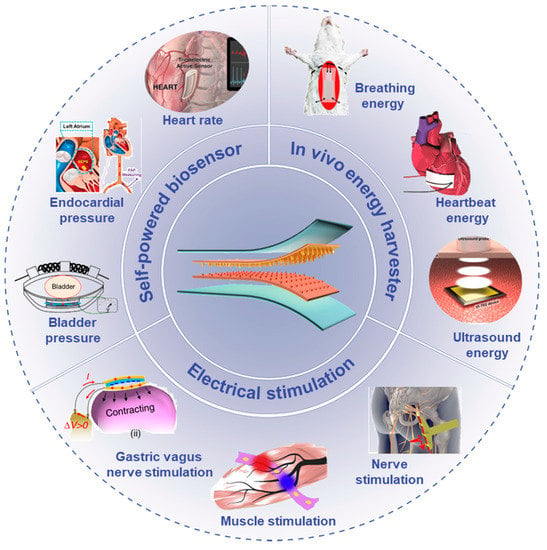The image showcases a detailed infographic centered on a "self-powered biosensor" involved in "in vivo energy harvesting" and "electrical stimulation." It features a prominent circular diagram bordered with blue dotted lines, segmenting into nine distinct sections, each labeled and illustrated with relevant icons. 

Starting from the top left and moving clockwise, the sections are as follows: 
1. "Heart rate" accompanied by a heart illustration.
2. "Breathing energy" with a corresponding image.
3. "Heartbeat energy" also depicted with a heart.
4. "Ultrasound energy" alongside its symbol.
5. "Nerve stimulation" illustrated accordingly.
6. "Muscle stimulation" with an illustrative depiction.
7. "Gastric vagus nerve stimulation" represented visually.
8. "Bladder pressure" with a relevant icon.
9. "Endocardial pressure" depicted accordingly.

In the center of the circle, the terms "self-powered biosensor," "in vivo energy harvester," and "electrical stimulation" are prominently displayed. Surrounding these terms is a vertical array of four ramp-like objects in green, yellow, orange, and another green layer, positioned one below the other. The diagram connects scientific concepts with visual elements to effectively communicate the functionalities of in vivo biosensors and energy harvesters.